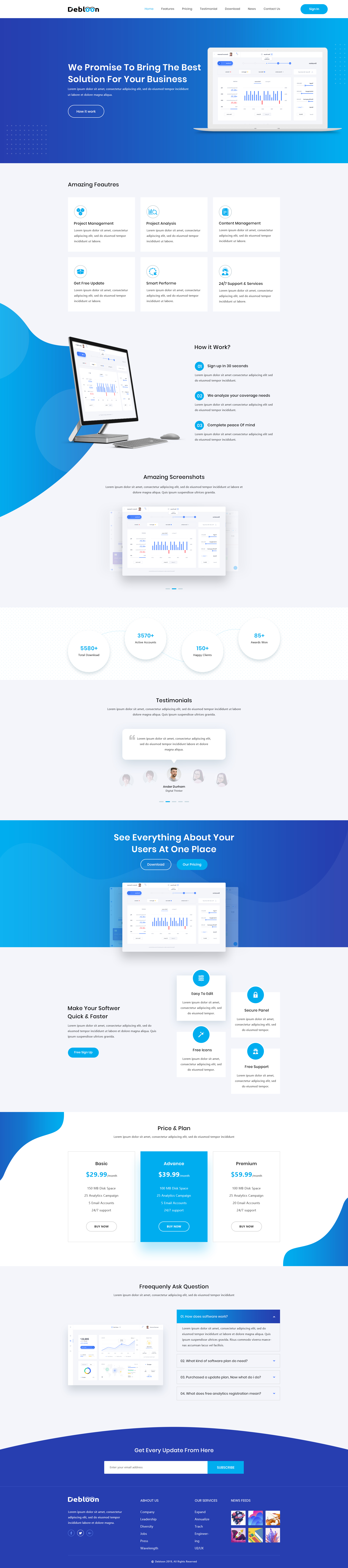A screen capture of an entire website, presented in a tall, scrolling image format. Due to the compressed nature of the image, the content appears very small. At the top of the webpage, there is a header featuring a graphic of a laptop displaying a software interface, accompanied by the phrase "We promise to bring the best solution for your business." Below the header are six small boxes, the contents of which are indistinguishable due to the image's size. 

Further down, there is a visual of an all-in-one workstation setup, comprising a screen, keyboard, and mouse, displaying the same software graphic seen earlier on the laptop. Beneath this, there are four buttons, though the text on them is too small to be read clearly.

Continuing to scroll, approximately the fourth or fifth page down, the text "See everything about your users in one place" is visible, alongside a repeated image of the software interface on a screen. At the very bottom of the page, the word "Debtoon" (spelled D-E-B-T-O-O-N) is displayed, surrounded by various clickable options.